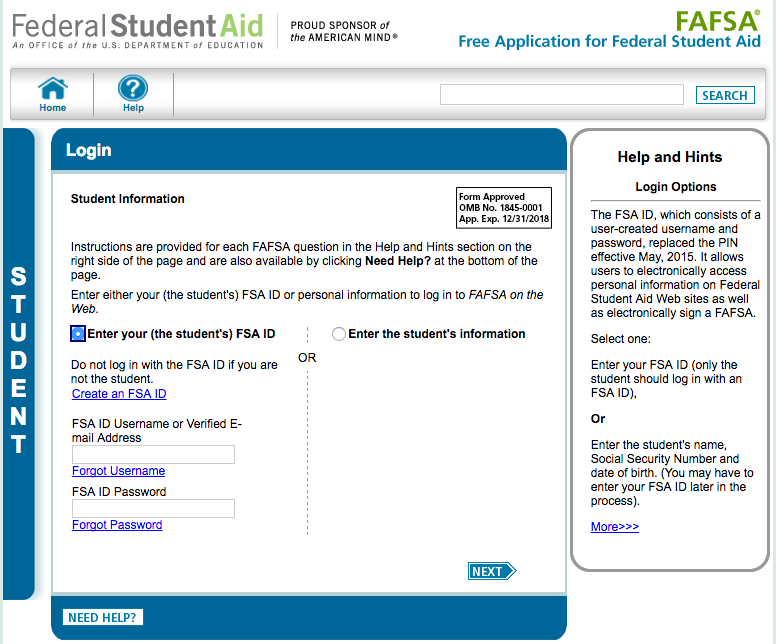The top left corner of the image features the text "Federal Student Aid," with the word "Aid" highlighted in green. Below it, in a smaller font, it reads "An Office of the U.S. Department of Education." To the right is the tagline "Proud Sponsor of the American Mind," with "AMERICAN MIND" written in all capital letters. On the far right, in prominent green all-caps, is the acronym "FAFSA" (F-A-F-S-A). Underneath, in blue text, it states "Free Application for Federal Student Aid," followed by a search bar.

To the left, there is a long blue line with the word "Login" written on it. Further left is a vertical blue line with the word "Student" written vertically. Beneath this, detailed student information and instructions are provided for each FAFSA question within the "Help and Hint" section on the right side of the page. Additional assistance can be accessed by clicking on "Need Help?" marked with a question mark.

Next to a blue square, there is the instruction: "Enter your (the student's) FSA ID" followed by a small circle option. In black text, it also reads "Enter the student's information." On the right side, within a vertical box, the headings "Help and Hints" and "Login Options" are displayed. Below this, an informational paragraph provides further guidance. It includes the text "Enter the student's name, Social Security Number, and Date of Birth," with a note in parentheses stating, "You may have to enter your FSA ID later in the process."